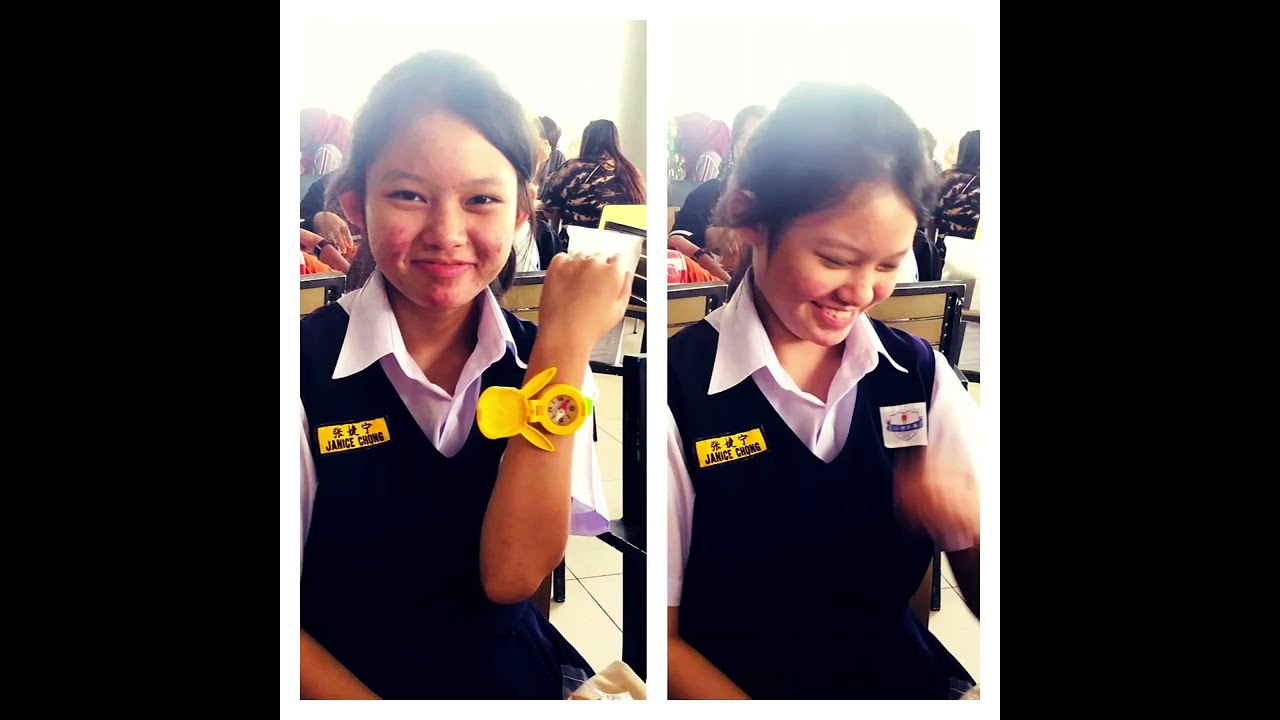In the image, there are two vertical photos of a young Asian girl, possibly of Chinese descent, who appears to be around 5 or 6 years old. She has long brown hair tied back in a ponytail and behind her ears, and she is wearing a school uniform consisting of a white button-down shirt and a dark blue vest sweater. On the left side of her vest, there is a yellow name tag with Chinese text at the top and the name "Janice Chong" in blue text below.

In both photos, the girl has noticeable acne on her cheeks and chin but maintains a bright and cheerful demeanor. In the left photo, she is smiling directly at the camera, holding up her left arm to display a yellow watch adorned with what appears to be a bunny motif. Her right arm is bent forward, and her posture suggests she is actively showing the watch to the viewer. In the right photo, she is looking down and away towards her arm, which has now become a motion blur, indicating she was in the process of moving it to look at the watch. 

The watch itself has a whimsical design reminiscent of a potted plant or a cartoon character, adding a touch of playfulness to her appearance. Behind her, a group of other children and possibly some teachers are gathered and sitting in a circle, providing context that this is likely a school setting. The background on the far left and far right of the photo is black, highlighting the girl as the central figure in the image.

Overall, the dual images capture Janice Chong in a candid and joyful moment, showcasing her exuberant personality while also providing context about her school environment.